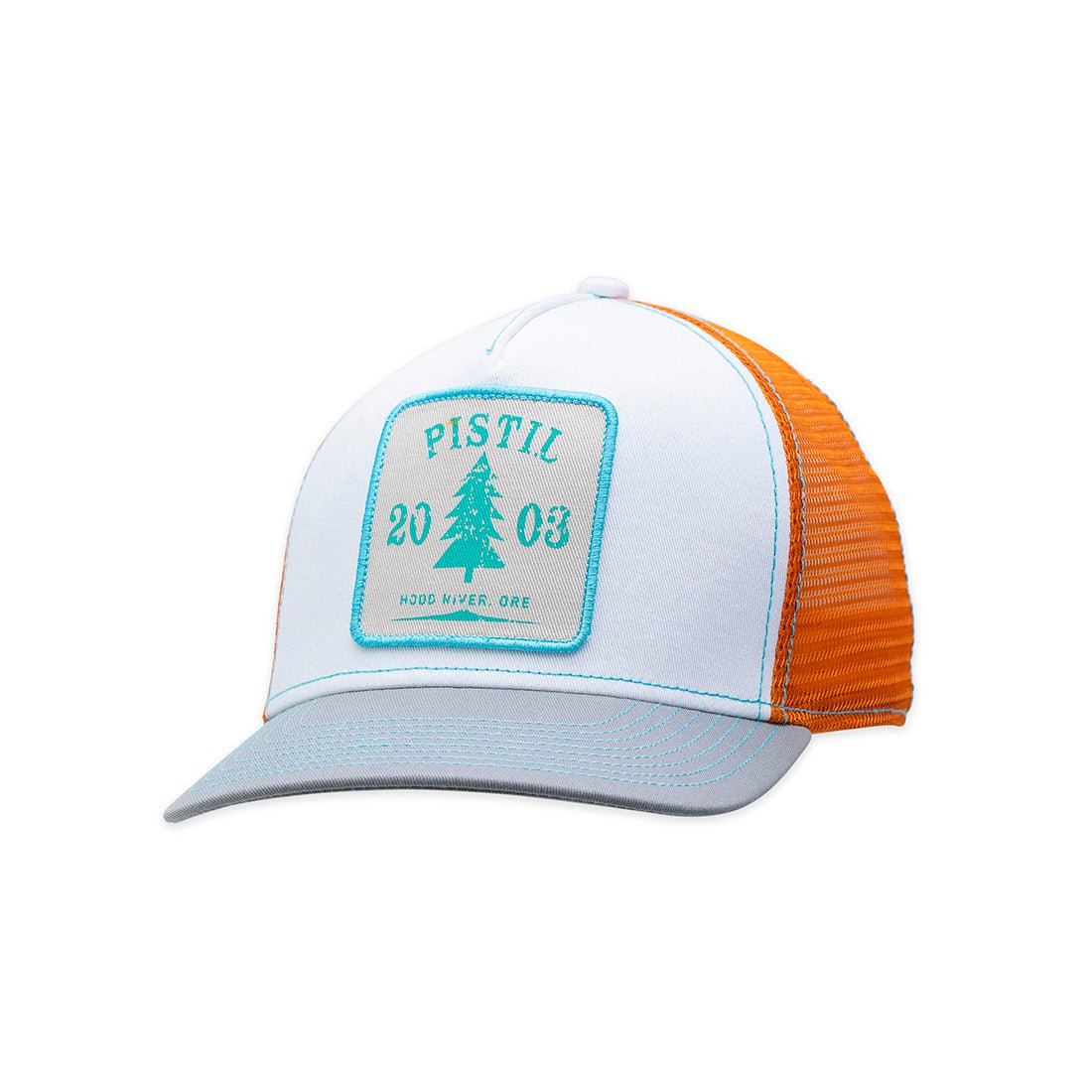This detailed image showcases a vibrant baseball cap placed against a solid white background. The hat's front panel is white with intricate turquoise stitching, while the back features bright orange mesh material, adding both color and texture. A white button sits at the top where distinct seams converge. 

At the center of the front panel, there's a distinct off-white square patch bordered with a thicker teal stitching. Inside the patch, the word "PISTIL" is prominently displayed in capital letters, followed by an evergreen tree design beneath it. To the left and right of the tree, the numbers "20" and "03" are written respectively, symbolizing the year 2003. Underneath the tree, the words "Hood River, ORE" are stitched in teal, followed by a small design in the same color.

The bill of the hat is light gray and features meticulous lines of turquoise stitching emanating from one side, stretching across the bottom and up the other side, creating a harmonious blend of colors and craftsmanship throughout the hat.